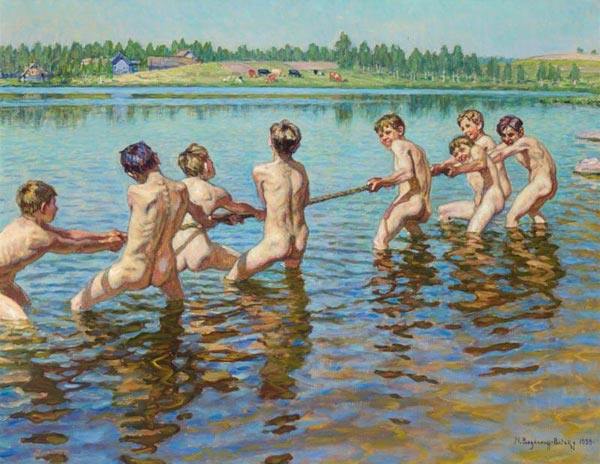This image is an oil painting set outdoors in a lake during the daytime, likely a replica of a famous work by Thomas Eakins. The scene depicts eight naked boys, around nine or ten years old, engaged in a spirited game of tug-of-war at the center of the image. Four boys line up on each side of the rope, with their spines and buttocks prominently visible. The water, brownish near their knees, reflects the vibrant green grass and blue sky peppered with white clouds. In the background, a field dotted with cows stretches out, flanked on the left by a house with a gabled roof and a brown barn, and on the right by lush, green trees. The landscape is tranquil, with more trees extending behind the house and barn. Faint text at the bottom appears to include "N-B-A-Z," possibly partly unreadable except for a discernible date, 1955, suggesting it is not the original painting.